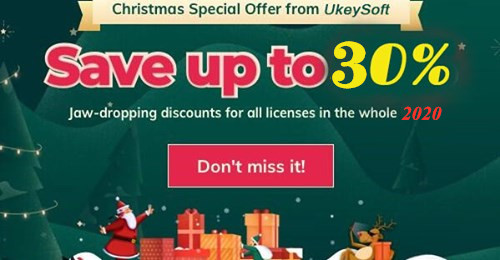This landscape-oriented promotional image from UKeySoft captures a festive Christmas Special Offer. The advertisement spans approximately twice its height and features a white, ribbon-like banner at the top with green text reading "Christmas Special Offer from UKeySoft." The majority of the background is a vibrant green, adorned with small, decorated trees and strands of festive lights.

In bold, large letters outlined in white, "Save Up To" is prominently displayed in pink, followed by "30%" in striking yellow. Beneath this, the text "Jaw Dropping Discounts For All License in Whole 2020" is positioned in white, with "2020" emphasized in red. A pink box with a white border below contains the enticing phrase "Don't Miss It" in white font.

The lower section of the image features charming Christmas-themed illustrations. These include a traditional Santa Claus in his red suit, a collection of 4-5 presents, and a hardworking elf dressed in green. To the right, a relaxed, cartoon reindeer sporting sunglasses and antlers reclines with an arm around a present.

Overall, this lively ad promotes UKeySoft's 30% discount offer, although the specific products or services provided by UKeySoft are not mentioned.